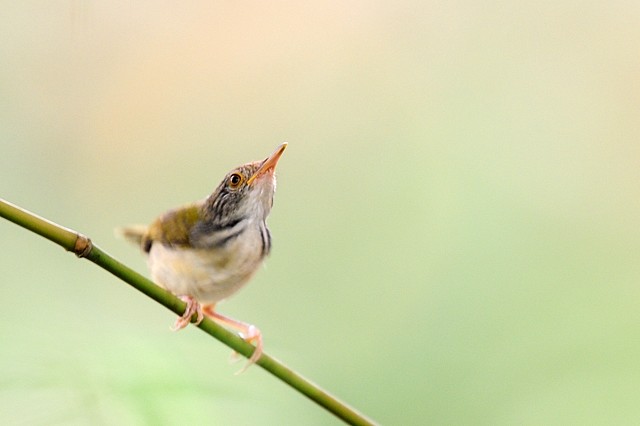This image features a detailed, zoomed-in photograph of a small songbird perched on a slender, light green twig that contains some brown coloration. The bird is positioned towards the bottom left corner of the image, facing slightly upward to the right, giving us a clear view of its intricate features. It has a white chest, brown and white feathers with hints of yellow, and a blackish-grey head with faint mottled stripes. Its beak is a tannish pink, and its feet are a pinkish-salmon color. The bird's eyes are brown, and we can observe one of its eyes clearly as its head tilts upwards, adding a sense of motion to the scene. The background is a soft, blurry gradient of green and light green, fading into a pinkish-orange hue in the upper left corner, which contrasts and enhances the sharp focus of the bird and the twig.